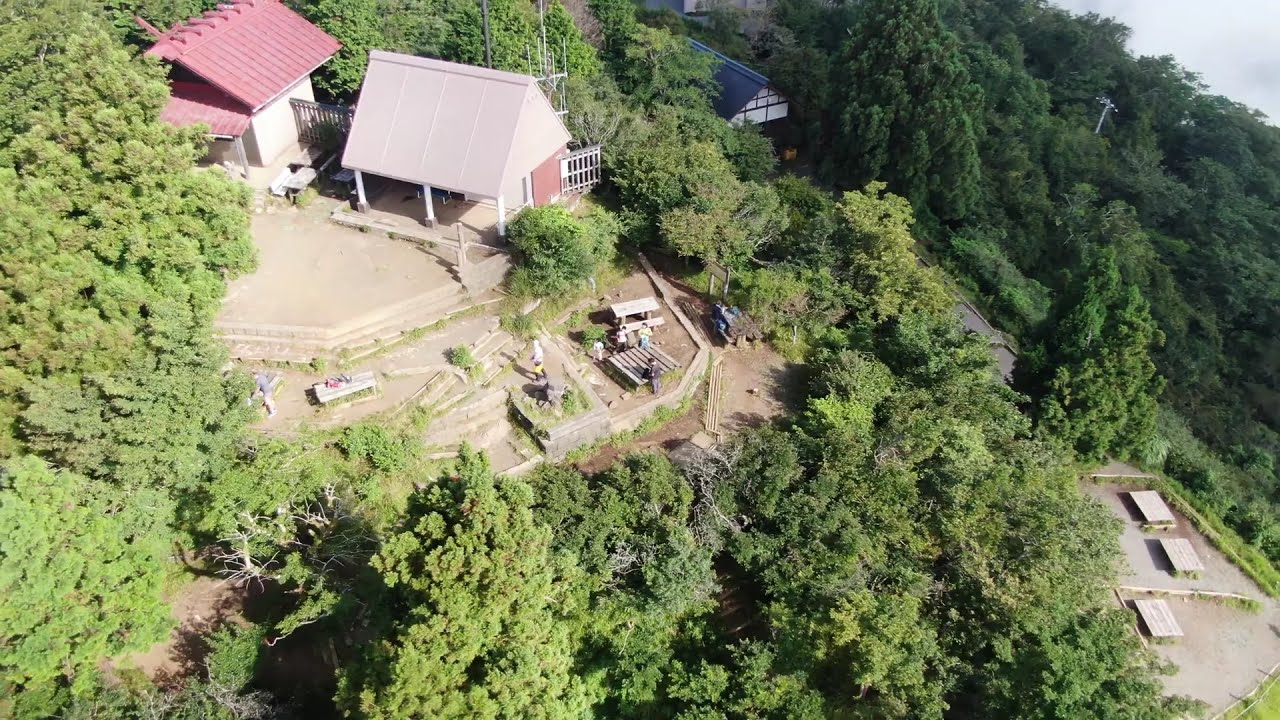The image depicts a bright, sunny wilderness area featuring a hillside surrounded by a dense array of trees. In the mid-right portion of the picture, there's a small clearing where sit two single-story houses: one with a triangular white roof and another attached house with a red roof, both made of light-colored stone. The landscape is slightly sloped, with various green trees and shrubs covering most of the ground. To the upper left, another house is visible, sporting a blue roof and white walls, while a hint of a blue-roofed building appears further in the background toward the center. Scattered around the houses are construction materials and some fenced areas. People are engaged in building activities with lumber in the open space in front of the houses, suggesting ongoing construction. The scene also includes evidence of potential landscaping or picnic areas, providing a multidimensional view of a lively and natural setting amidst a forest environment.